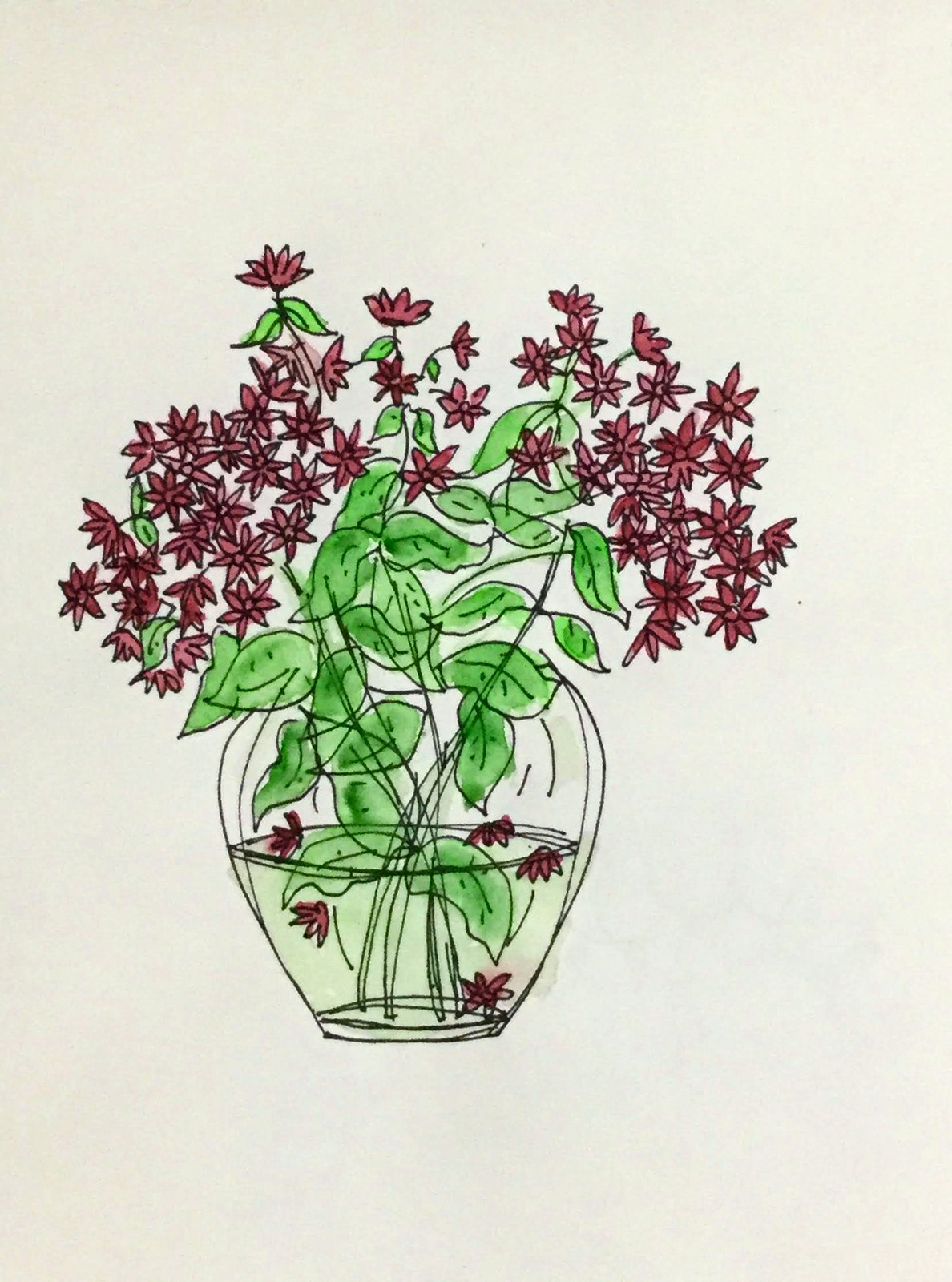This artwork depicts a beautifully rendered vase of flowers, centrally positioned against a simple, tan background, which may be the natural color of the paper. The vase is transparent, resembling glass, allowing a clear view of the green-tinted water within. This subtle tint suggests the natural leaching of color from the stems and leaves. Inside the vase, a few fallen blossoms float on the water's surface, adding a touch of realism. The arrangement features a lush collection of green leaves that provide a verdant base, rising upward to support an array of delicate, reddish-purple flowers. Each small blossom appears to have approximately five petals, contributing to the intricate and detailed nature of the piece. The flowers are more densely clustered on the right and left sides, with a slightly sparser distribution in the center, creating a balanced but dynamic composition. Overall, the painting captures the essence of a fresh and vibrant floral bouquet with elegant simplicity.